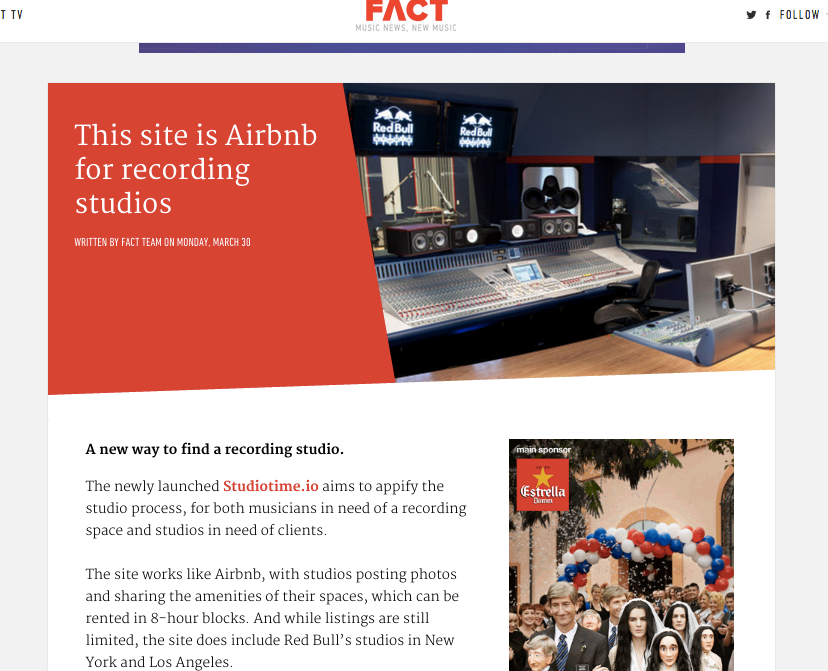The image displays a webpage from the Fact Music News New Music website. The upper right corner offers options to follow the page on Twitter or Facebook. In the upper left corner, there's a logo featuring "T-TV" with a color scheme of red, white, blue, and black text against a contrasting background. Also in the upper left corner, there is a red background with white text. 

The central focus of the page is an article titled "Airbnb for recording studios," written by the Fact Team and published on Monday, March 30th. To the right of the title is an image depicting music-making equipment in a recording studio. Below this image, the text describes a new platform, studiotime.io, which aims to streamline the process of finding and booking recording studios. The site functions similarly to Airbnb, allowing studios to post photos and detail their amenities. These spaces can be rented in eight-hour blocks. Though the listings are currently limited, notable studios like Red Bull Studios in New York and Los Angeles are already featured.